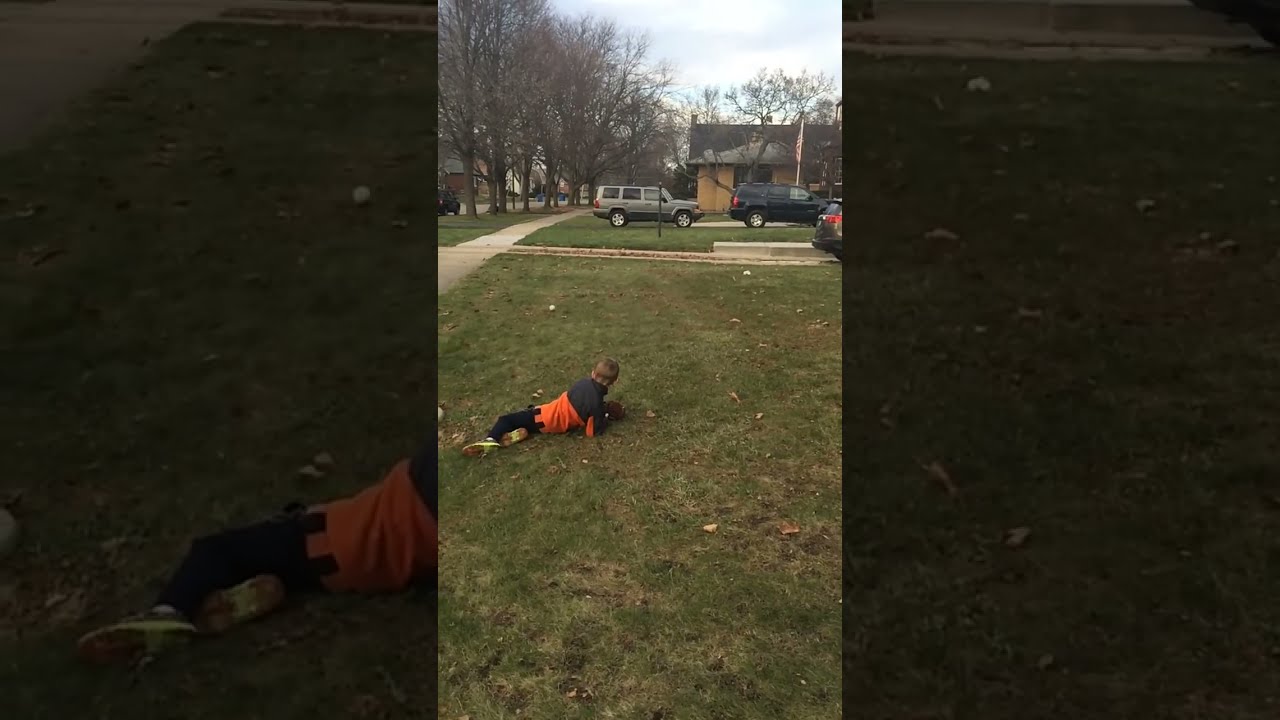In the image, a young boy, around six to seven years old, is poised to catch a baseball in a typical American suburban neighborhood. He has short blonde hair and is smiling eagerly, holding a black baseball mitt high in his left hand with his right hand also raised, capturing an action shot from the perspective of the ball thrower. The boy is dressed in a gray and orange sweater and black pants, standing in a green and brown lawn scattered with autumn leaves. The backdrop features a sidewalk, bare trees lining the street, a few SUVs—a blue one and a gray one—parked in driveways, and various cars further down the road. A tan house with a brown roof is also visible. The baseball, white with red stitching, is suspended mid-air against a blue sky with wispy white clouds, heading towards the child. The scene underscores a peaceful, chilly day in fall or winter within a quintessential American neighborhood.